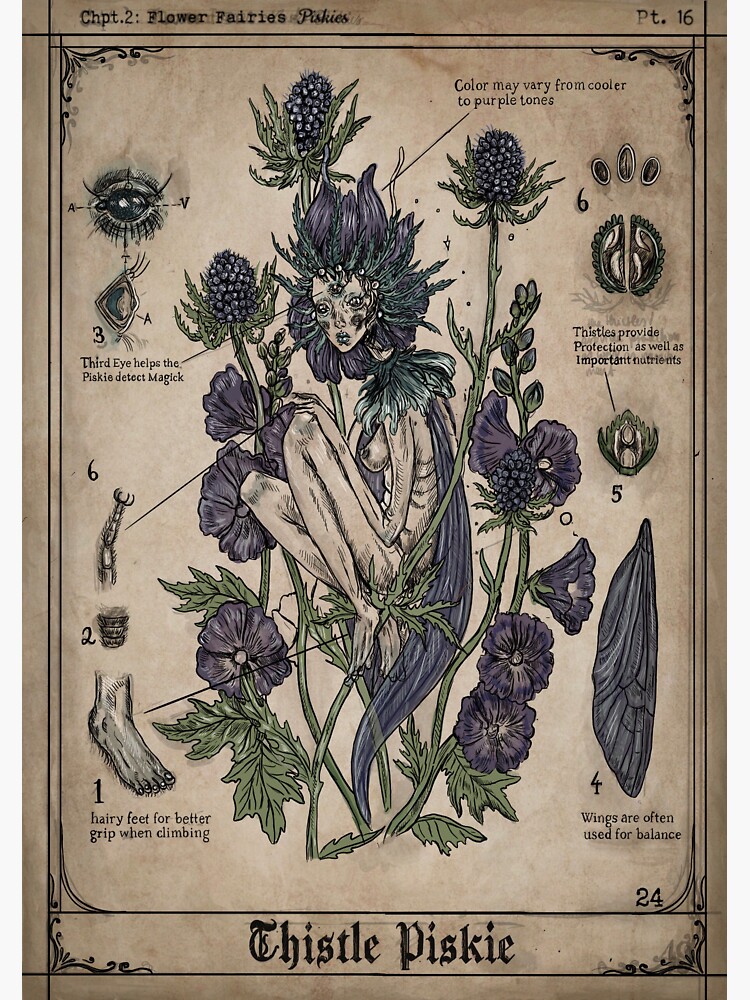This detailed illustration from an old-fashioned field guide, specifically page 24 of the Flower Fairies chapter, showcases a thistle pixie, a whimsical and delicate creature from fairy tale fantasy. The artwork features a petite, nearly naked humanoid figure, crouched with her knees up near her, nestled amidst a cluster of dark purple and green thistles and flowers. The pixie's head and face are framed by these floral elements, and she wears a distinctive green fringed collar made of leaves. Her unique features, such as her hairy feet for better grip, a third eye on her forehead to detect magic, and wings used for balance, are meticulously numbered and explained in the illustration. The pixie's body, a plant-like beige tone, contrasts against the cream background, while the thistles, known for protection and nutrients, add to the fantastical ambiance. The color scheme of the image ranges from cooler to warmer purple tones, and the thin lines framing the artwork give it an art deco feel. This illustration captures the ethereal essence of the thistle pixie, blending botanical elements with magical lore.